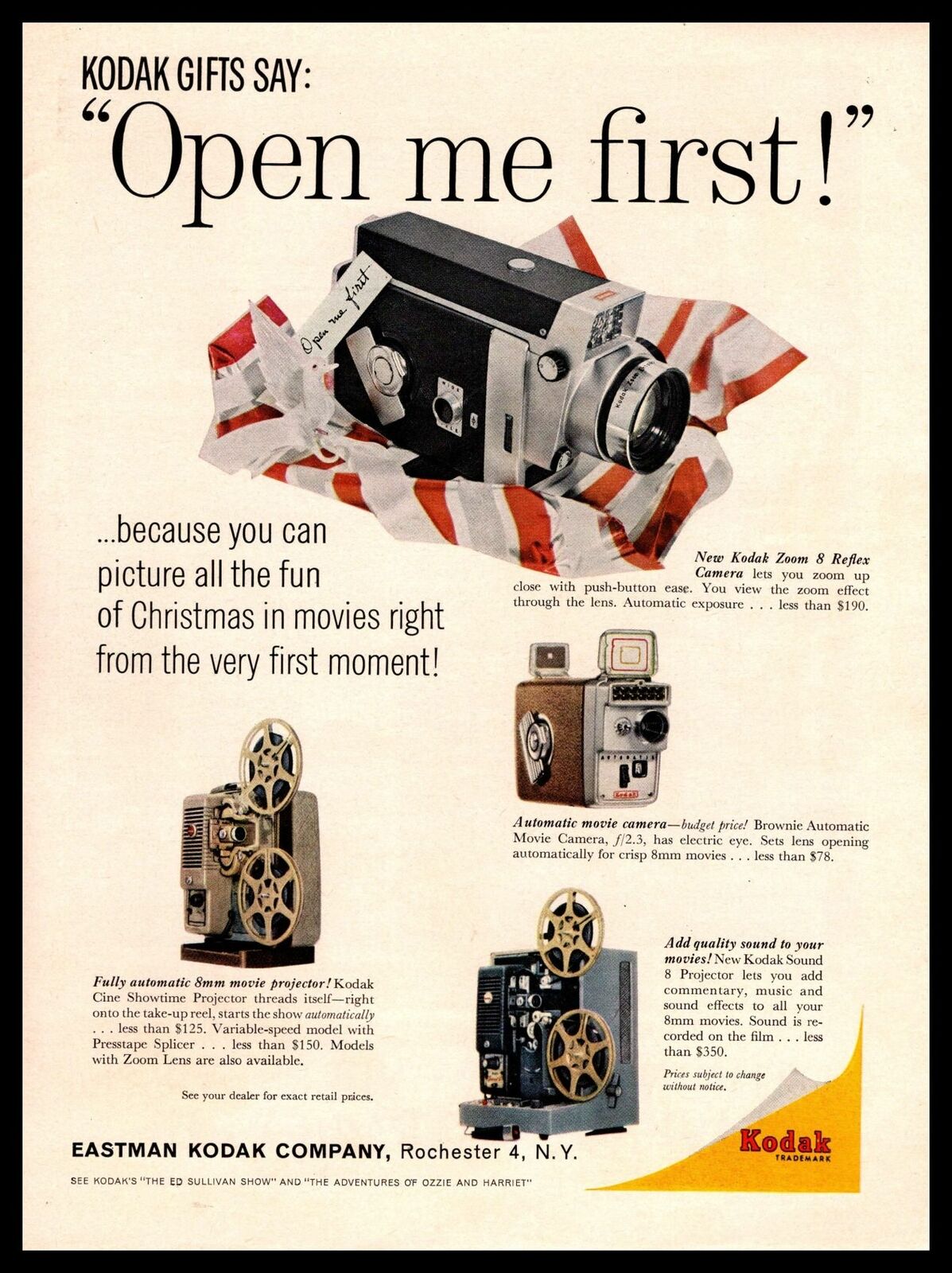The image is a vintage advertisement, likely from a magazine, featuring a white background bordered by a narrow black frame. At the top left, in dark letters, it reads "Kodak gifts say:", followed by the phrase "Open me first!" in larger, quoted text. This headline emphasizes the excitement of capturing Christmas memories from the very first moment. Below this text, there is a black camera partially wrapped in red and white paper, as if freshly unwrapped. To the left of the camera, the ad continues with the phrase, "Because you can picture all the fun of Christmas in movies right from the very first moment." Lower down, the advertisement showcases additional vintage equipment: a brown movie camera and two projectors, possibly from the 1950s or 1960s, complete with manual film reels. These projectors, likely 8mm or 16mm, suggest a focus on home movie making. The bottom right corner features the Kodak logo within a yellow triangular shape with red font. Further text mentions the Eastman Kodak Company of Rochester, New York, though much of it is too small to read clearly. The page appears to be curling up at one corner, adding to the nostalgic feel of the ad.